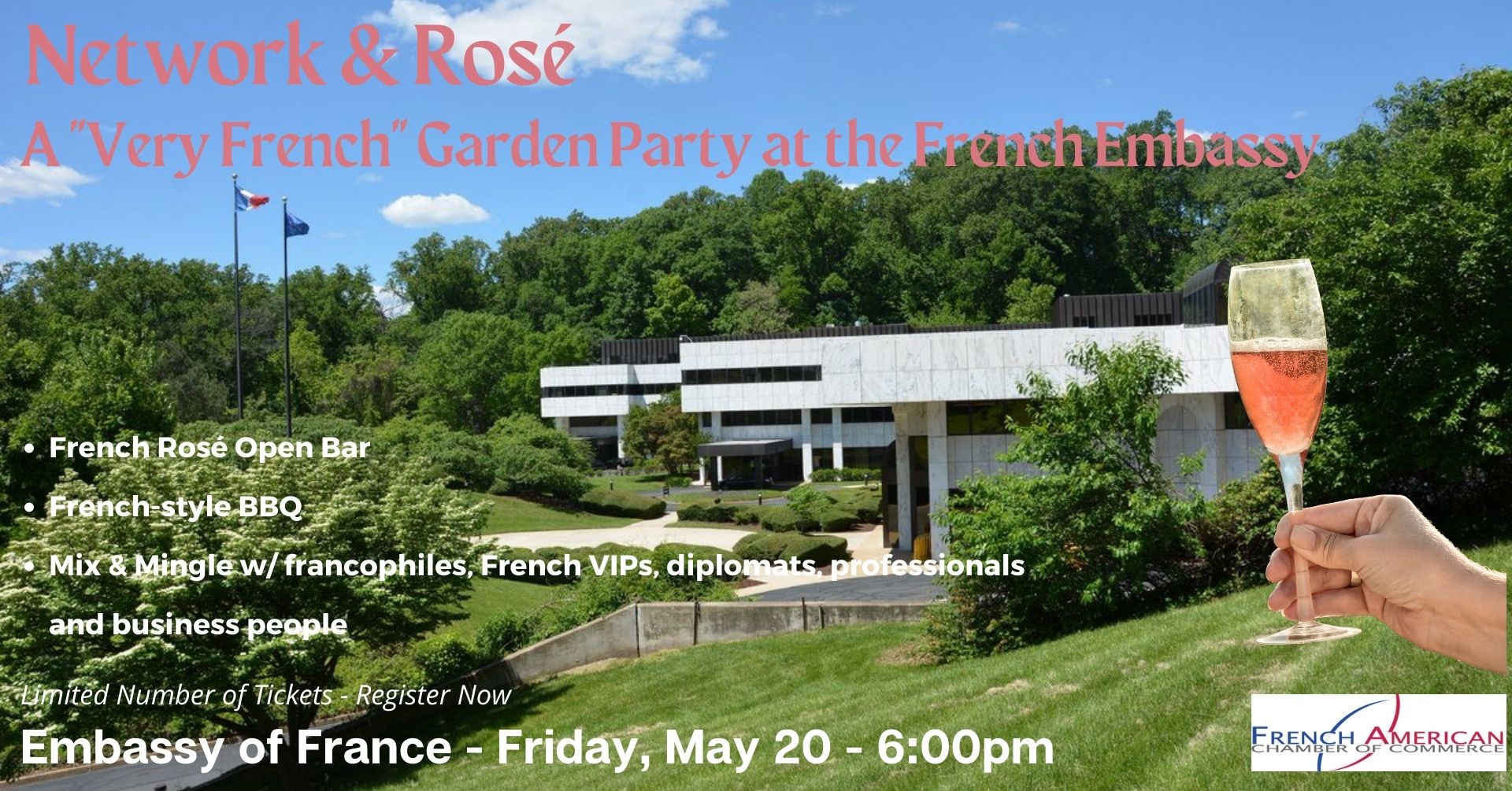This image depicts an advertisement crafted from a daytime photograph of an outdoor scene, featuring a background of a blue sky with white clouds and a row of green trees beneath it. Centered in the image is a modern white building with two flags in front of it. On the right edge, a hand is prominently holding a champagne flute filled halfway with rosé wine. On the top left, text in pink reads "Network and Rosé," with an asterisk over "Rosé." Below, it declares, "A very French garden party at the French Embassy." Additional details on the left side of the image articulate the event's features: "French Rosé open bar," "French style barbecue," and the opportunity to "mix and mingle with Francophiles, French VIPs, diplomats, professionals, and business people." At the bottom left, there is a note in small print stating, "Limited numbers of tickets. Register now." Finally, in larger white print at the bottom, it details, "Embassy of France – Friday, May 20 – 6 p.m." Additionally, on the right, a white rectangle contains the text "French" in blue, "American" in red, and "Chamber of Commerce" in black beneath it, with a subtle background logo.